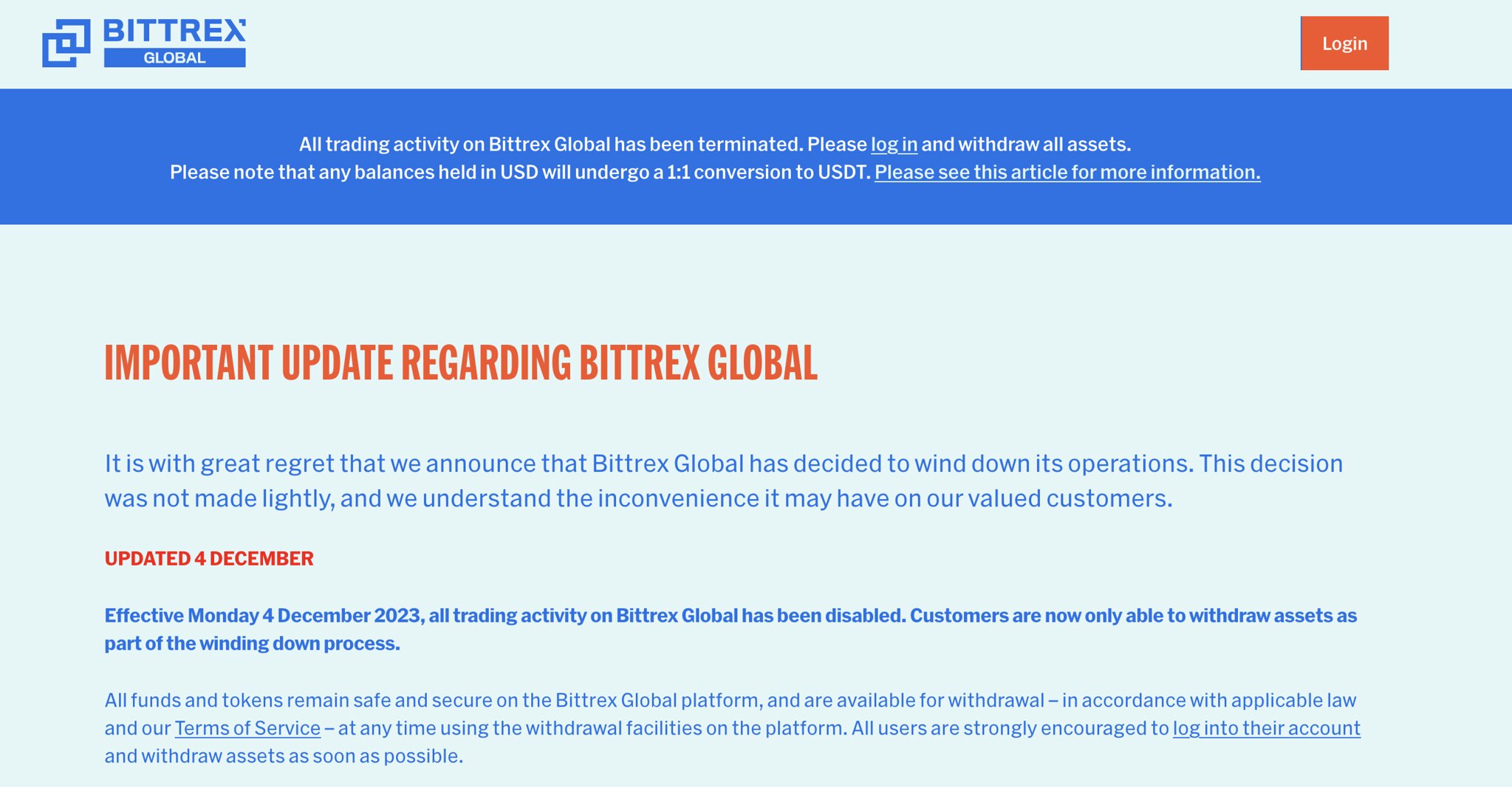The image is a screenshot of Bittrex Global's login page, featuring a light blue background with a blue logo in the upper left corner, consisting of two interlocking squares followed by the text "Bittrex Global." In the upper right corner, there's an orange rectangular login button with white text that says "Log In." Below the login button, a prominent blue horizontal bar spans across the top of the page, with white lettering announcing: "All trading activity on Bittrex Global has been terminated. Please log in and withdraw all assets. Please note that any balances held in USD will undergo a 1-to-1 conversion to USDT. Please see this article for more information." Underneath this bar, a light blue section features an "Important Update" in large orange letters regarding Bittrex Global. The announcement states that the company is winding down its operations, a decision made with great regret and understanding of the inconvenience to customers. It concludes with a note that the information has been updated for December 4th, 2023.